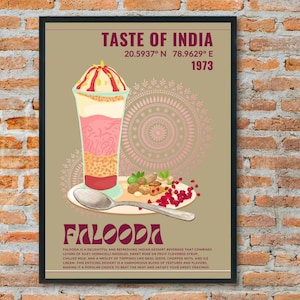The image is an advertisement for an event called "Taste of India," which appears to be a festival celebrating Indian cuisine and culture. The advertisement prominently features the word "Faluda" in large marine letters and includes specific geographic coordinates (20.5937° N, 78.9629° E) and the year "1973." The background has a light brown color and the design includes a pink swirling pattern.

The central image showcases a multi-layered smoothie-like dessert placed on a plate. The layers from bottom to top are red, orange with brown dots, pink, white, tan with brown dots, and a top layer resembling white ice cream with red syrup. Accompanying the dessert are cherries and green or brown circular fruits, all arranged on a plate with a silver spoon. The entire photo is mounted on a brick wall with round bricks and a light fixture in the middle. The bottom part of the advertisement contains five sentences written in small marine-colored letters, which are not easily readable.